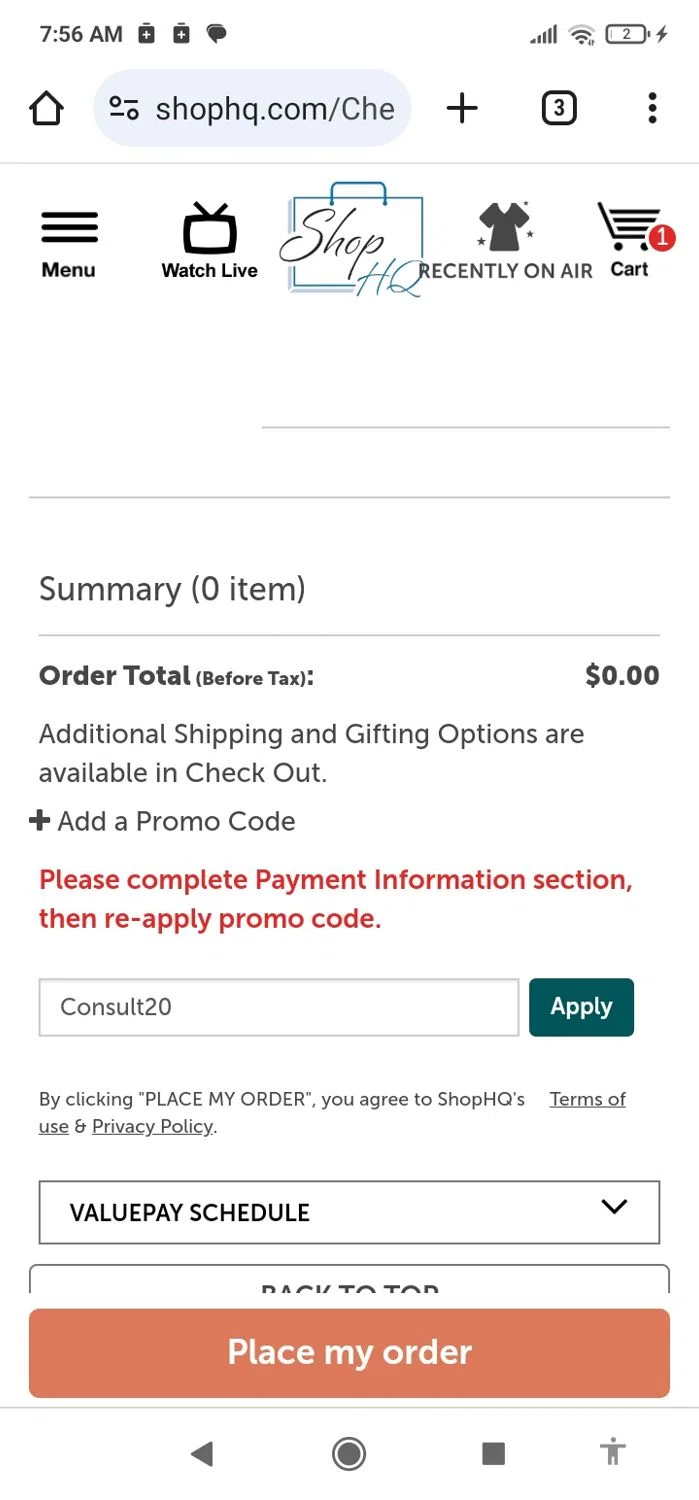This mobile screenshot from Shop HQ’s online shopping cart showcases an overview of the checkout process. At the top, it prominently displays "Summary" with "0 items" in parentheses, indicating an empty cart. Directly underneath, it states "Order total," also marked as zero dollars before tax. It further notes that "Additional shipping and gifting options are available in checkout," accompanied by a plus sign for expanding options. 

Adjacent to this, users are prompted to add a promo code, with instructional red text underneath explaining, "Please complete payment information section, then reapply promo code." The input field beside this text shows the promo code "CONSULT20" already entered, with an 'Apply' button in teal color next to it.

Below these prompts, in very small font, is a disclaimer stating, "By clicking Place My Order, you agree to Shop HQ's Terms of Use and Privacy Policy." Additionally, there is a "Value Pay Schedule" button featuring a dropdown menu option, followed by an eye-catching orange "Place My Order" button in white letters, ready for finalizing the purchase.